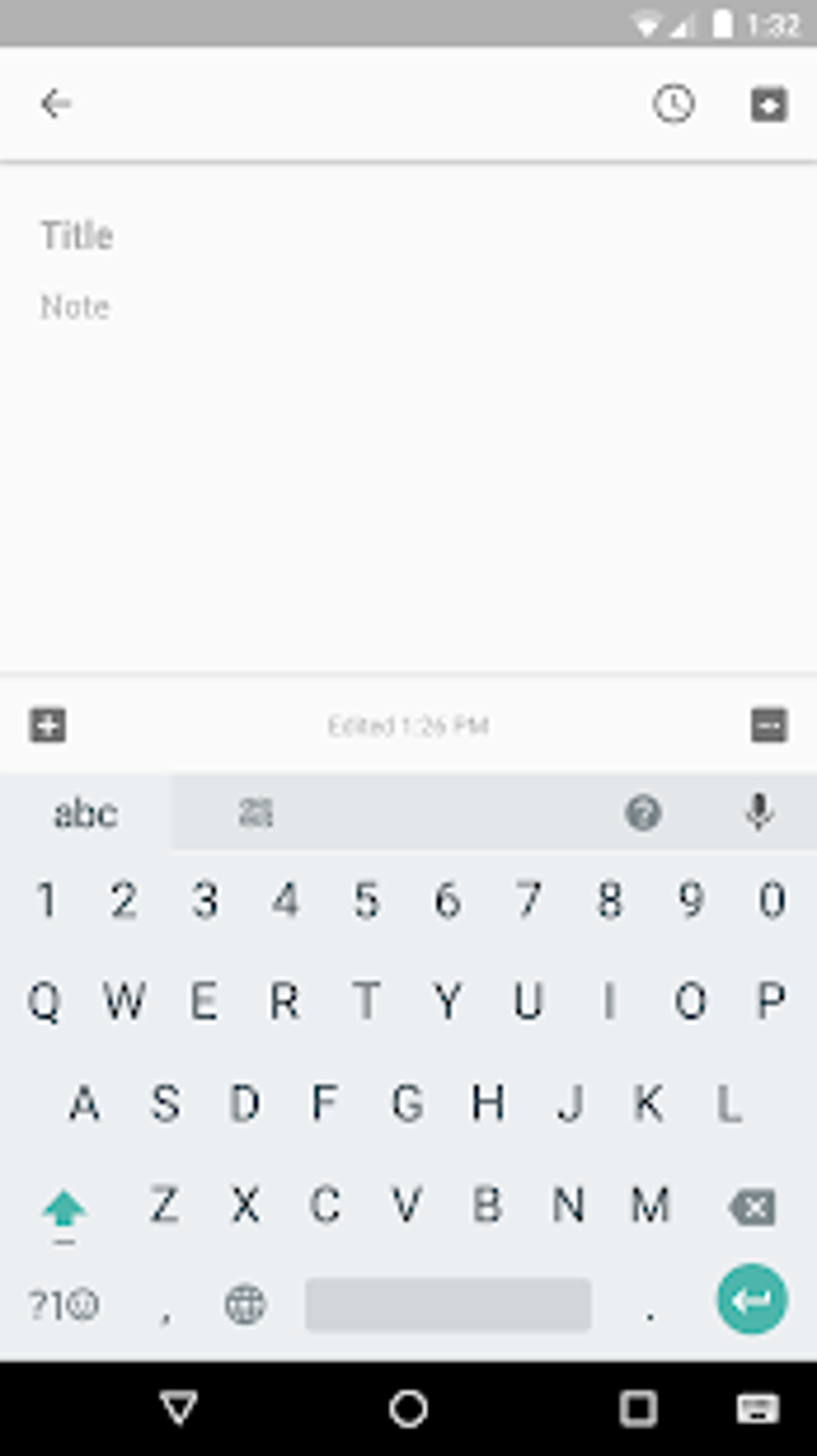This image captures the screen of a cell phone with intricate details. At the top, a long, skinny gray rectangle stretches across the screen. On the left side, it is empty, while the right upper corner displays several status icons: a Wi-Fi symbol, a cellular signal bar, and a fully charged white battery icon. The time, 1:32, is also visible in this top section.

Below the top bar, there's an arrow pointing left, followed by a clock icon and a plus sign enclosed in a box. A faint gray line separates this area from the next section, which features the word "Title" in gray print. Directly underneath, the smaller word "Note" appears, and the rest of this section is blank.

Further down, another faint gray line introduces an input area, demarcated by a gray region where text can be entered. At the top of this section, "ABC" is visible, along with a blank line containing a microphone icon and a question mark for voice input. The virtual keyboard below is laid out with the numeric keys 1 through 0 on the first line, followed by the alphabet letters arranged on subsequent lines.